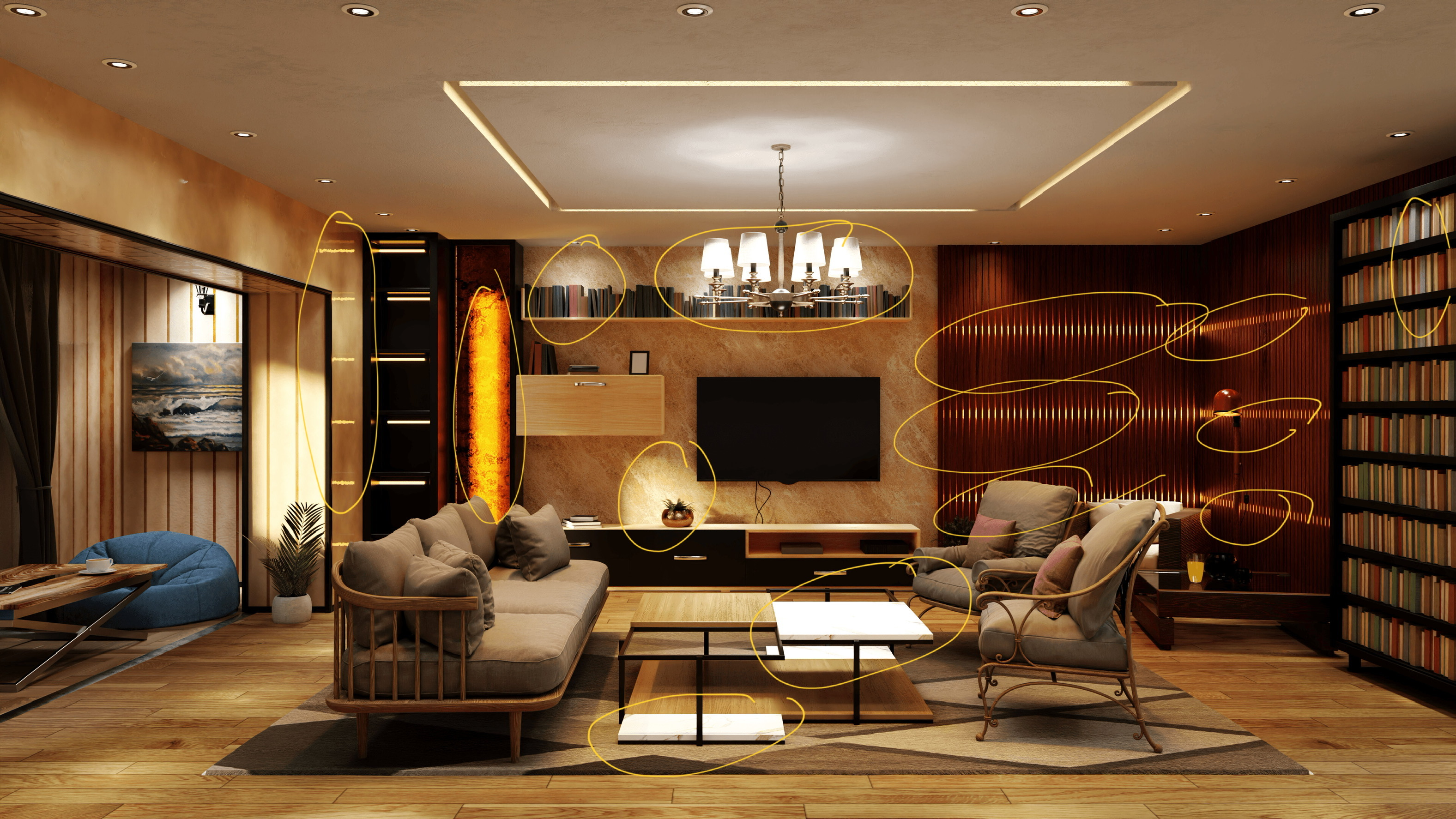The image depicts a cozy living room area, possibly a basement room or a library within a house or hotel, characterized by a warm and inviting atmosphere. The room features a large brown couch and two tan chairs arranged around a set of coffee tables. The floor is lined with beige wood, adding a natural feel to the setting. A prominent geometric rug in various shades of brown and tan, designed with triangles, covers the floor beneath the furniture.

In the background, there is an extensive shelving unit, painted in different shades of red and black, filled with books, which adds a sense of depth and scholarly ambiance to the room. A flat-screen TV is mounted against a tan wall, flanked by the shelving unit. A corduroy beanbag and a potted plant occupy a cozy corner, adding a touch of comfort and greenery.

The ceiling has a recessed design painted in white, featuring drop-down lighting and a glass fixture with multiple conical covers, ensuring that the room is well-illuminated. Notably, several objects in the picture, including the light fixtures, shelving units, and various items on a long desk, have been circled in yellow, suggesting their importance or relevance within the context of the room. There is also a decorative picture, whose specific details are unclear, adding an artistic touch to the setting.